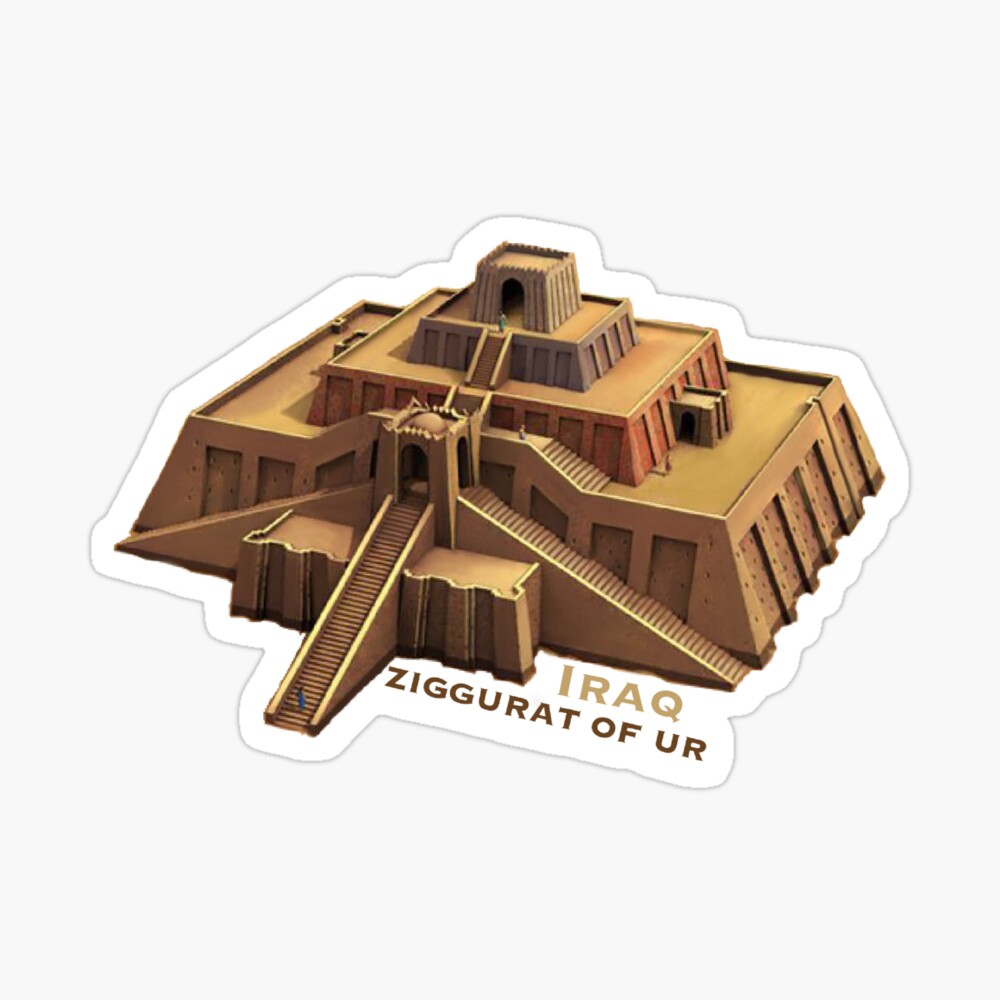This detailed image depicts the Ziggurat of Ur, a grand Neo-Sumerian structure located near Nasiriyah in present-day Iraq. The ziggurat, carved from sandstone or potentially wood, stands prominently with its mustard-brown hue against a gray background. The structure showcases four distinct, progressively smaller levels reminiscent of a pyramid's stepped design. The lower levels feature windows around the perimeter, though the interiors are obscured. At the base, three grand staircases ascend to the first elevated level, offering entrances from the front, left, and right sides. This level is encircled by a walkway, leading to stairs that climb to the third floor, which also features a surrounding walkway. A final set of stairs leads to the topmost level, crowned by a small square with an archway opening. The presence of a tiny figure emerging from this top entrance accentuates the monument's immense scale. The caption "Iraq Ziggurat of Ur" is inscribed on the image, further identifying the historical and geographical significance of this monumental edifice.